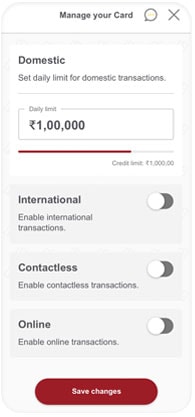Here's the cleaned-up and detailed caption:

---

The screenshot features a mobile banking application interface. At the top, the header reads "Miniature Card," accompanied by a chat bubble icon with three yellow dots, likely indicating support or assistance features, and an 'X' button for closing. Below the header, there's a box labeled "Domestic," offering the option to set a daily limit for domestic transactions, which appears to be set at $100,000 (however, the exact currency symbol is unclear, displaying as 1,00,000). A "Credit Limit" is also specified, showing the same value as the daily limit. Further down, there are three toggles: one for enabling international transactions, which is currently switched off; another for enabling contactless transactions, also switched off; and a third for enabling online transactions, again switched off. At the bottom of the screen, a prominent red button labeled "Save Changes" is visible, suggesting users can save any alterations made to their transaction settings.

---